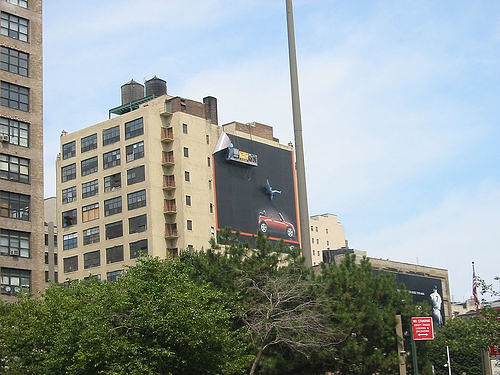This image captures the side of a 5 to 6-story building, primarily characterized by its black facade. Prominently displayed on the building is a billboard depicting a person seemingly falling from the sky into a red convertible. The advertisement's company origin is indistinguishable. In the foreground, lush green trees add a touch of nature to the urban setting. At the lower right corner, beneath the billboard, there is a red and white sign. Adjacent to this area is a smaller building with an image of a baseball player wearing number 7. To the left of the scene, a larger building with numerous windows completes the cityscape.